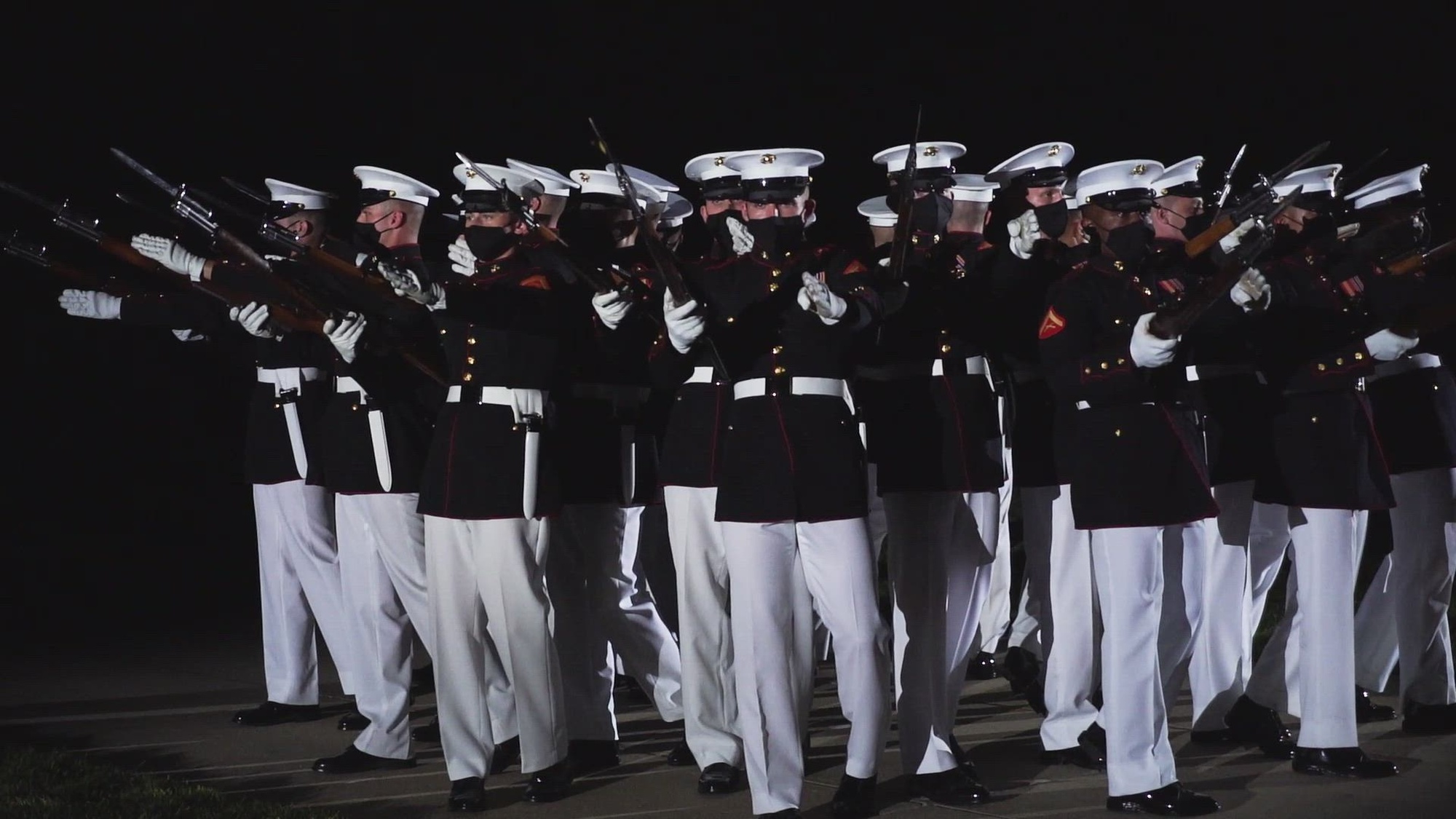The image is a detailed, color photograph taken at night, characterized by a dark background that deepens around the edges and bottom. The main subjects of this photograph are a troop of U.S. Marines, dressed in their formal dress uniforms, which comprise black tops with white belts, white pants, white gloves, and white caps bearing an emblem. They are all wearing black face masks, likely a precaution during the COVID-19 pandemic. The Marines are organized in a march-like formation with those at the front facing the viewer and others on each side facing outwards, either left or right. Each Marine holds a rifle, many with bayonets attached, reminiscent of those used in ceremonial salutes at military funerals. A figure in the foreground appears to be giving directions, adding to the sense of regimented yet slightly disarrayed military order. The image embodies the style of photographic representational realism, capturing the solemnity and precision of the Marine Color Guard.